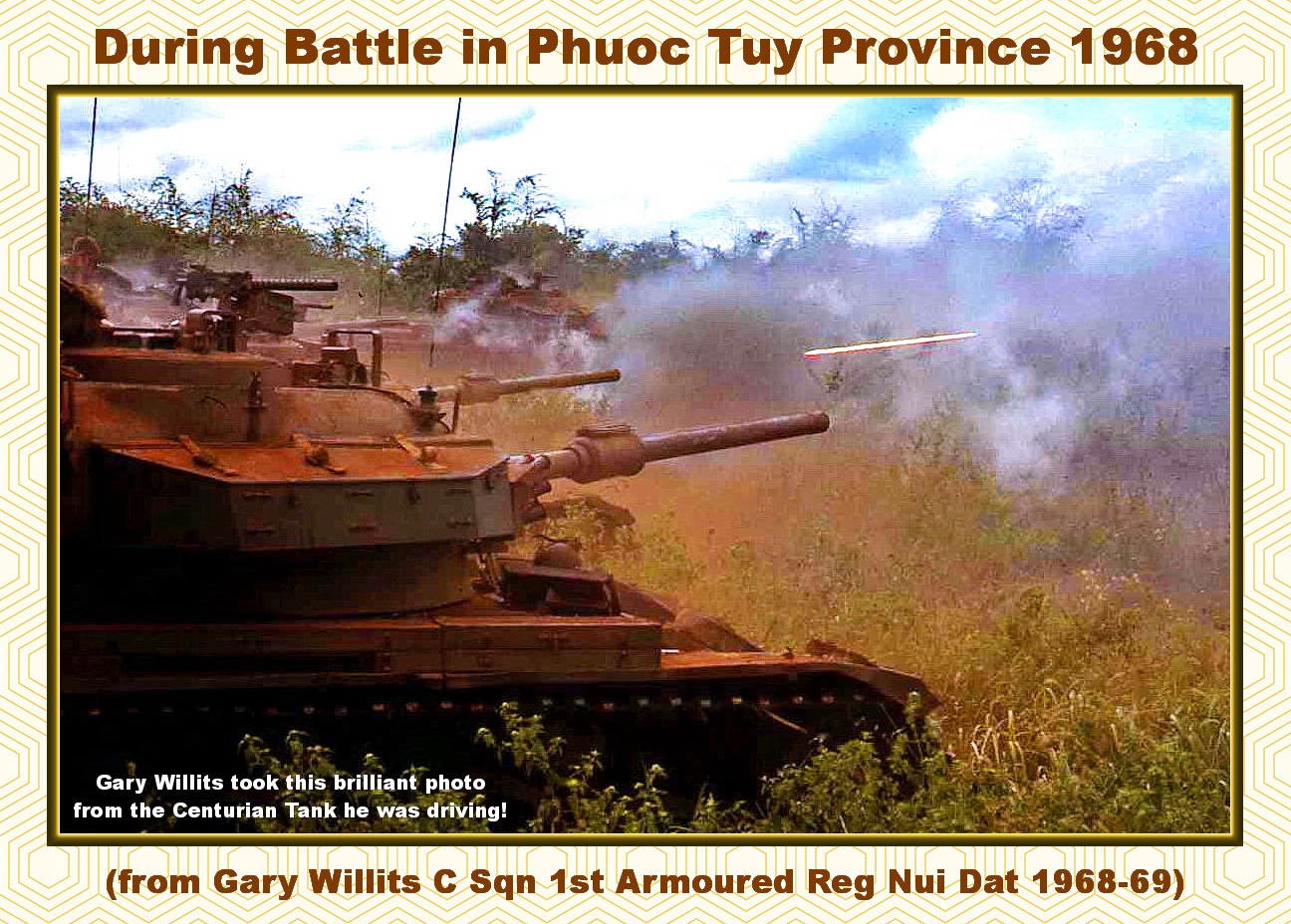The picture, surrounded by a light yellow geometric border with a hexagon pattern, vividly captures a battlefield scene during the Vietnam War. A brown text across the top border reads "During Battle in Phuoc Toi Province 1968," emphasizing the historical context of the image. The photograph, which has a striking black and yellow border, depicts a bright day with some clouds in the sky.

In the foreground, a row of four or five Centurion tanks is positioned on the left side of the image, firing towards the right. The intense action is evident with a lot of smoke billowing from the tanks' cannons towards the brush and trees on the right. A tracer shell is visible amidst the onslaught, adding to the dramatic intensity of the scene. Tall grass and dense vegetation can be seen in the background, though no people are visible.

At the bottom left corner of the photograph, white text states, "Gary Willits took this brilliant photo from the Centurion tank he was driving." Below the photograph, more brown text specifies, "(From Gary Willits, C-Squadron 1st Armored Regiment, Nui Dat 1968-69)," further accrediting the image.